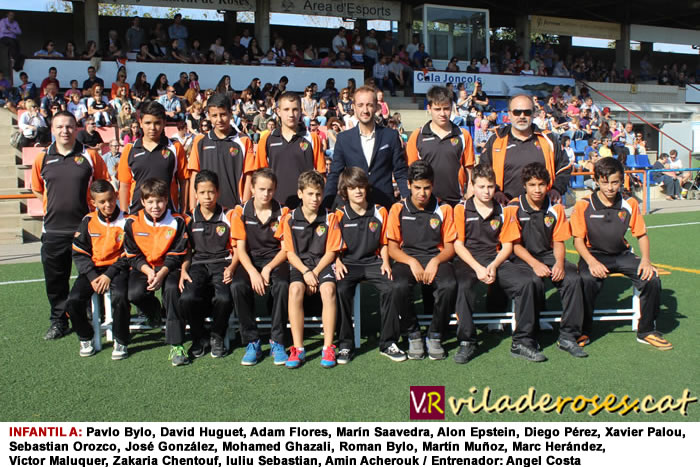This image is a photographic representation of a youth soccer team, captured outdoors in a green field during the daytime. The team consists of a dozen boys, mostly wearing black jerseys with orange sleeves, and they appear to be around 13 to 14 years old. Most of them are in black pants, with one boy in shorts. They are seated and standing in two rows, with the front row sitting on a bleacher and the taller boys and their coaches standing behind them. Behind the boys is a line of adults, mostly wearing the same black and orange jerseys, except for one man in the middle who is in a sports jacket. The group appears to be diverse, with most members being people of color, while the central sports jacket-wearing man and two others flanking him appear to be white. In the background, bleachers filled with spectators can be seen. The word "CHEALACONCOIS" is printed on the stands, and the bottom right-hand corner of the image features the text "VRVILADEROSES.CAT" with a caption underneath that reads "INFANTILA". Additionally, the names of the children are listed in Spanish below the photograph.